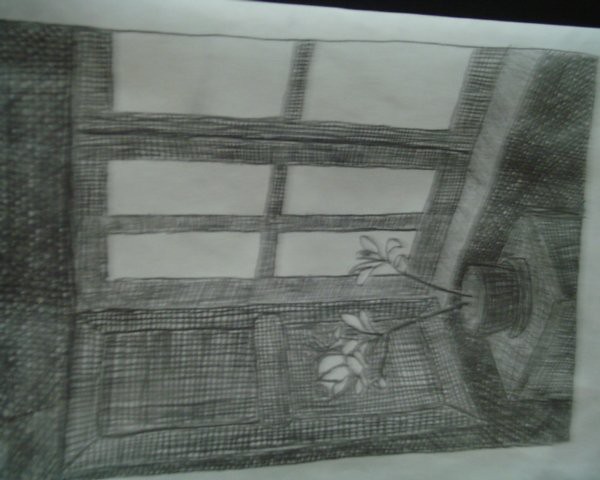This is a detailed pencil drawing on white paper, although the image itself is blurry and slightly unfocused. The scene is viewed from a side perspective and has been turned sideways, giving it a horizontal orientation. The drawing depicts a small square table with a planter on top, holding two flowers -- one primarily leafy and the other featuring what appears to be an open rose. The pot and table are intricately shaded. Behind the table, there is a window letting in sunlight, framed by a wooden shutter on the left side. The window's frame has separations forming a cross in its center, and above the window, a heavily shaded crosshatch pattern is visible. The walls around the window are also shaded in dark pencil tones, enhancing the depth and contrast of the scene. The entire drawing is set against a black background, further highlighting the white paper and the meticulous details of the artwork.